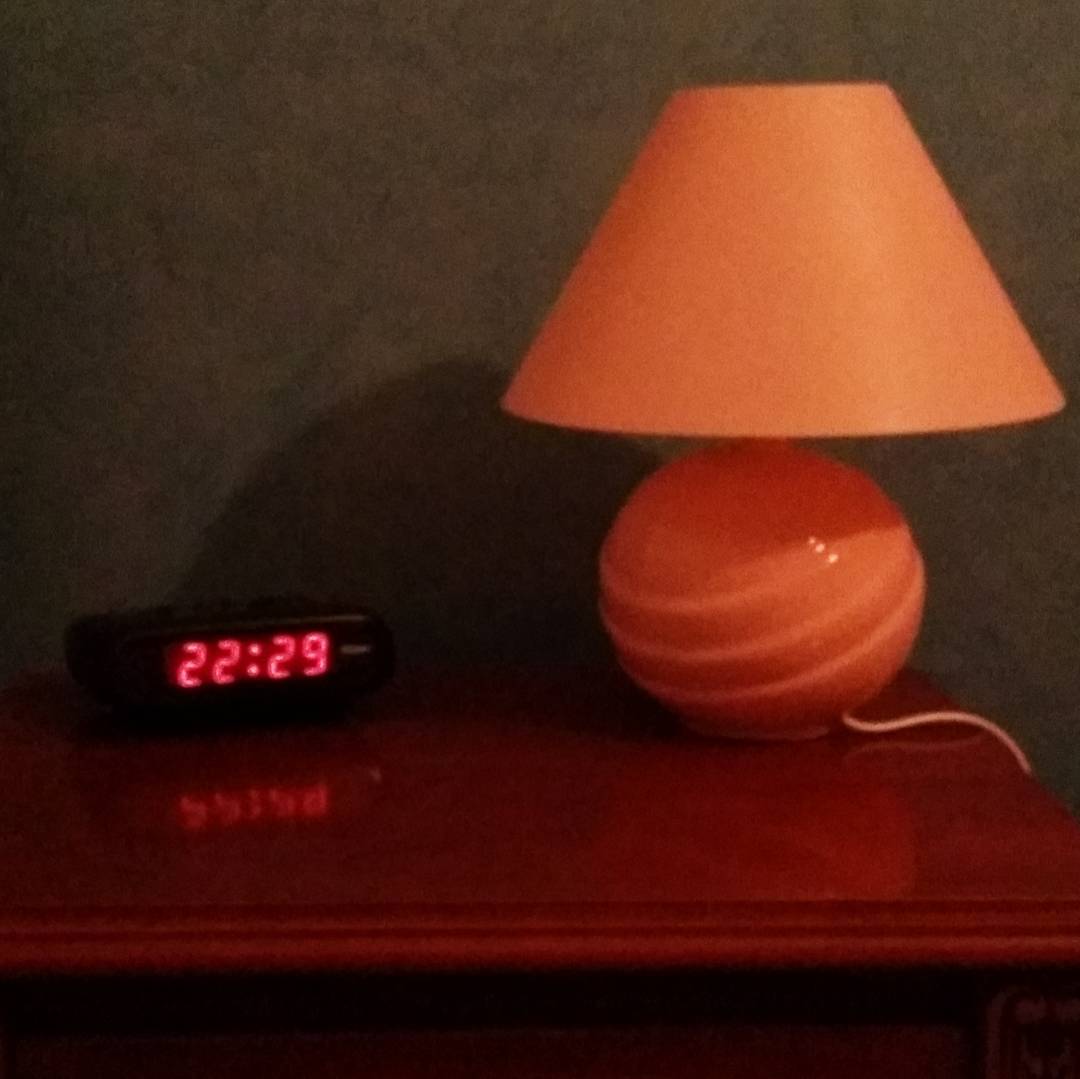The image depicts a well-polished, deep brown wooden nightstand situated in a dimly lit room with a gray, brownish-greenish wall in the background. On the left side of the nightstand is an old digital alarm clock with a black casing and red digital numbers displaying 22:29 in military time, its reflection subtly visible on the shiny surface of the nightstand. To the right is a distinctive spherical lamp with a glossy, orange base featuring sculpted ridges. The base connects to a slightly lighter, yellowish-orange lampshade that emits a soft glow. A cable can be seen extending from the bottom of the lamp's base, adding to the intricate details of this cozy, serene setting.